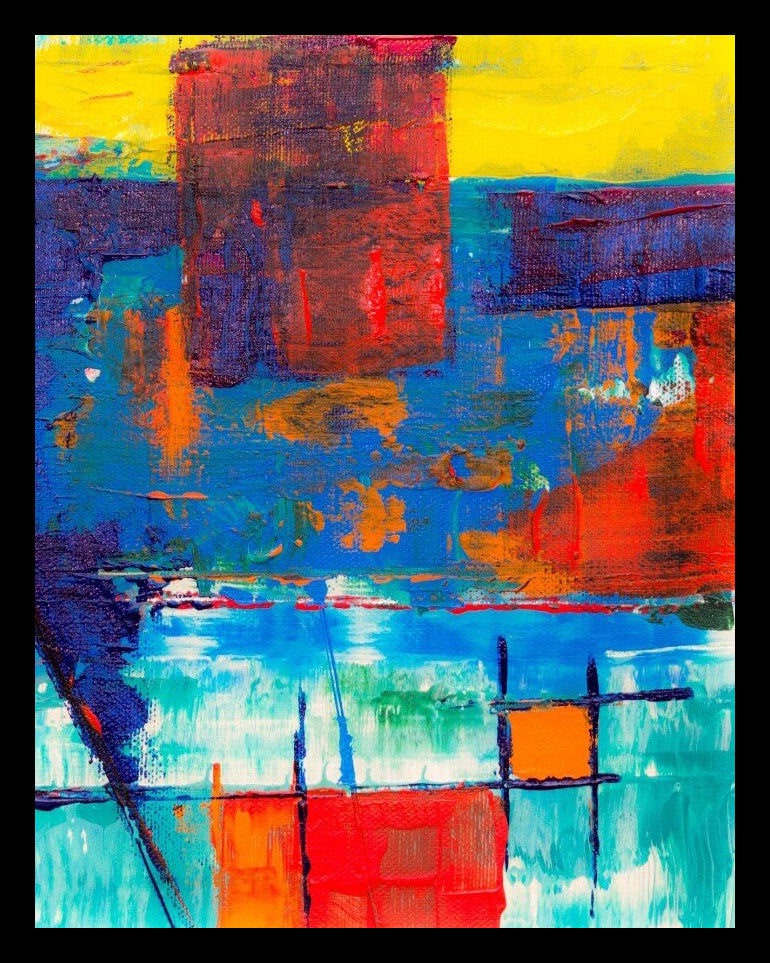This photograph captures an abstract modern art painting, outlined with a distinct black border, creating a striking frame for the vivid colors within. Dominated by a high-contrast and limited color palette, the painting primarily features blue, red, and orange, with subtle blending that introduces hints of green and cream. At the very top of the canvas, a bold stripe of yellow stands out as the only use of this color. Near the top left, there is a hand-painted red square, intermingled with darker blue shades to form a muddy texture. Swatches and splashes of orange are scattered centrally without any discernible shape. The lower half of the canvas transitions to an aqua blue, distinct from the lighter blues above, and hosts another red square, accompanied by intersecting blue lines creating a smaller orange-filled square. The right side displays vivid red patches, while the left shows a gradient from dark to light blue, blending towards green and cream hues. The painting’s contemporary allure lies in its bold, irregularly shaped blocks and the way its colors seem to bleed and blend together, inviting a personal interpretation from its viewers.